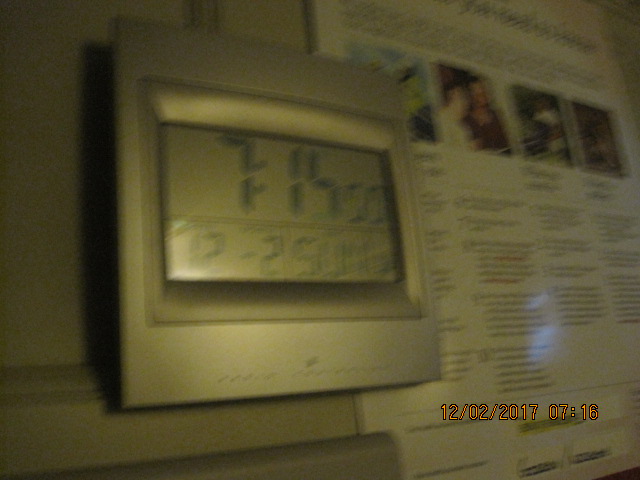This photograph captures a digital wall clock mounted on a gray wall. The clock has a silver plastic frame and a clear plastic face displaying large black digits. The primary time displayed is 7:15:50, accompanied by a secondary set of numbers below: 12-5, though further characters are obscured. The clock face is divided into two sections by a horizontal line, separating the top two-thirds from the bottom third. Additional smaller digits, difficult to decipher, are present in this lower section. In the bottom right-hand corner of the photograph, a date and time stamp reads: 12-02-2017 07:16. Adjacent to the clock, a poster with four images is partially visible, featuring predominantly black and white text with occasional red accents.